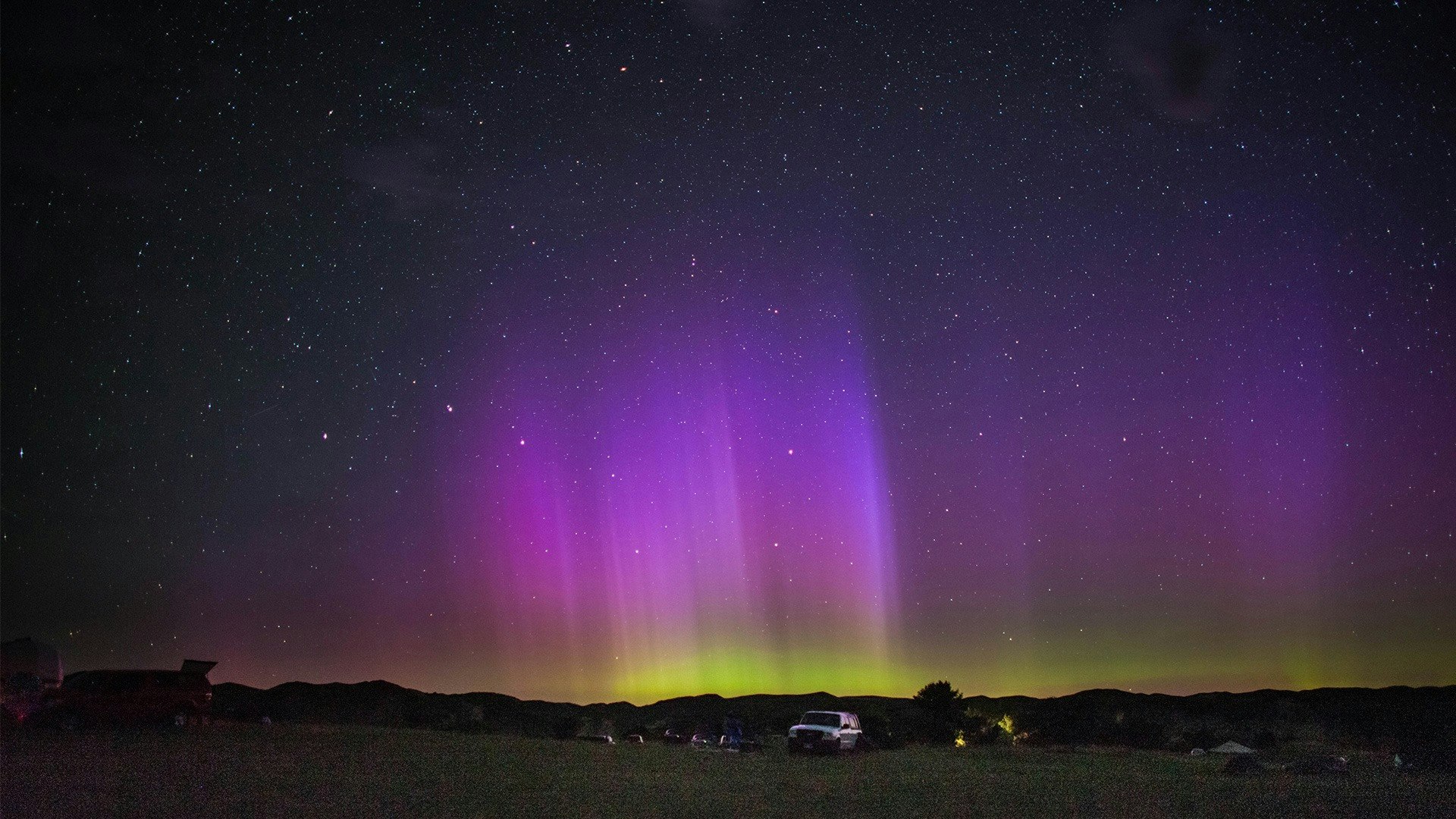This captivating night scene prominently features the ethereal dance of the northern lights across the sky. At the top, a myriad of stars twinkle in various hues, predominantly white. As your eyes move downward, the sky bursts into streaks of vibrant purple, creating a vertical, uneven, and choppy pattern reminiscent of the aurora borealis. Towards the horizon, a soft yellow glow hints at either a tinge of light pollution or a distant sunset.

Below this celestial display, the landscape is dark but discernible. Silhouettes of hills or mountains stretch across the image from left to right, their outlines barely visible in the night. Towards the center of the scene, a vehicle—possibly a truck or SUV—sits far off in the distance, while to its left, another silhouette suggests the presence of a van. Nestled near this central vehicle appears to be a rudimentary camping area, where indistinct objects are arranged in a loose semi-circle.

On the ridge in the foreground, the ground seems smooth and perhaps grassy despite the darkness. Here, several more cars or possibly some tents or small buildings can be faintly seen, indicating that people might be camped out, captivated by the luminous spectacle overhead. The entire image is bathed in a mystical aura, with the northern lights casting a mesmerizing purple and yellow glow upon the night sky.